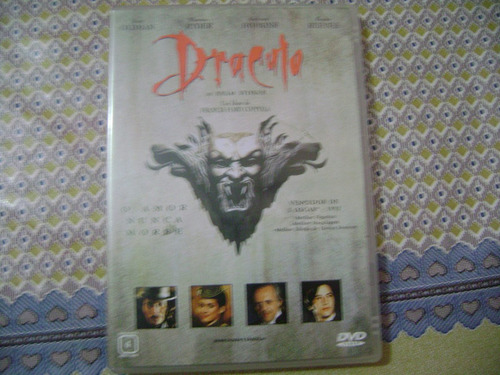In the center of the image is a DVD case for Bram Stoker's Dracula. The DVD features cover art akin to the promotional poster for the film. At the top, in red, blood-dripping text, is the title "Dracula." The case prominently displays an evil Dracula face with long fangs in the center. Along the bottom, four small screenshots of the film’s actors—Keanu Reeves, Winona Ryder, Anthony Hopkins, and Gary Oldman—are framed inside boxes from right to left. The background color of the DVD cover is largely gray. At the top, though blurry, the actors' names are listed. Situated atop a fabric believed to be a tablecloth, the DVD case is surrounded by an intricate pattern. The tablecloth transitions from a diamond pattern with off-yellow, gray, and blue colors to blue hearts with gray interiors towards the bottom, eventually turning green. The bottom left corner of the DVD case shows a regional symbol, and the DVD logo appears in white at the bottom right corner.